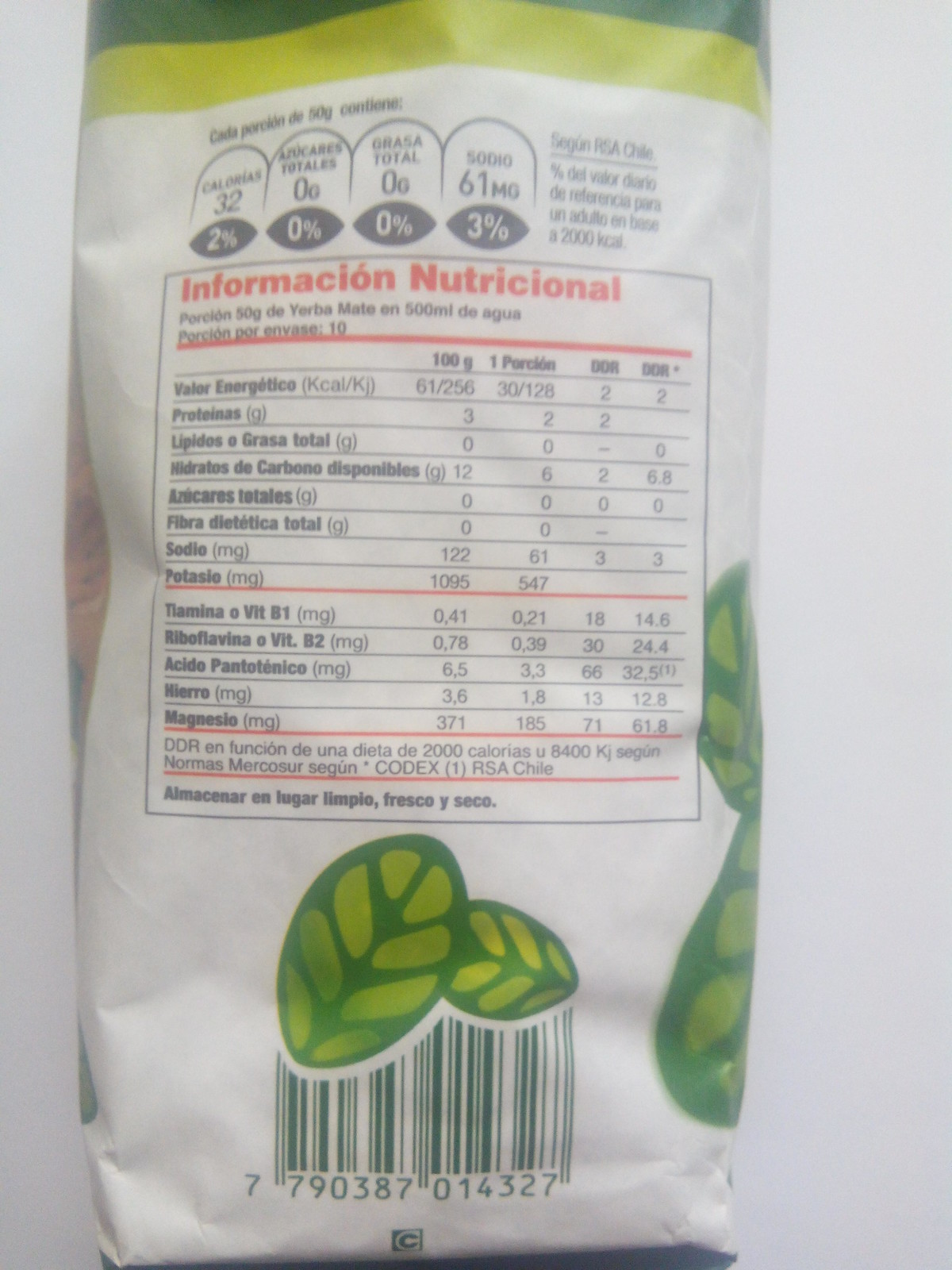The image showcases the back of food packaging designed to resemble a white paper bag adorned with leaf graphics. The top portion prominently features the "Información Nutricional" section, which is presented in red font, indicating that the nutrition facts are listed in Spanish. Below this header, the standard nutrition chart is displayed, outlining key nutritional elements such as sodium, potassium, various vitamins, and proteins, each accompanied by their respective values. Further down, two green and yellow leaf illustrations add an aesthetic touch to the packaging design. At the very bottom, a barcode is neatly positioned, completing the informative and visually appealing layout.